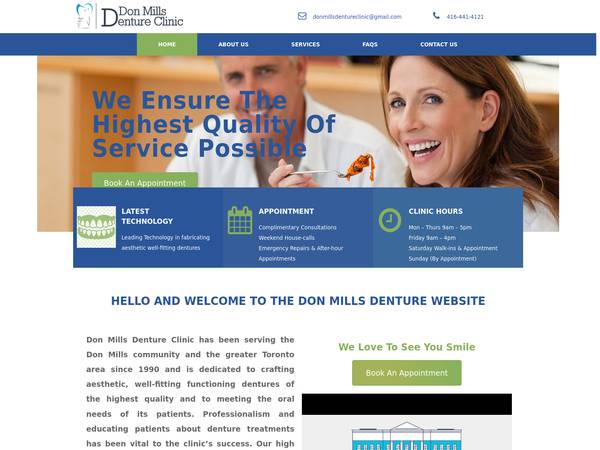**Caption: Don Mills Denture Clinic Website Interface (Screenshot)**

The screenshot captures the interface of the Don Mills Denture Clinic website. At the top within a white bezel, there's a symbolic tooth design with a cyan-blue upper half and a gray lower half featuring squiggly lines. Right below this, separated by a gray line, is the bold blue text displaying the clinic's name: "Don Mills Denture Clinic." 

Adjacent to this text, the contact email is provided as "donsdentureclinic@gmail.com," accompanied by a blue envelope icon. Alongside is a blue phone icon with the contact number "416-441-4123."

The dark blue bezel at the top showcases several clickable menu options. The currently selected option, "Home," is highlighted with a green rectangle. The other unselected options in white text include "About Us," "Services," "FAQs," and "Contact Us."

The main content area features an image of an older man with gray hair dressed in a lab coat, standing beside a woman with shoulder-length brown hair and blue eyes, who is smiling while holding a fork with orange pasta. Both individuals have light skin.

Overlaying this image is the text: "We ensure the highest quality service possible." 

Below this text, a dark blue rectangle is presented, above which a smaller green rectangle contains the call-to-action text "Book an Appointment." The dark blue rectangle includes a symbol of teeth, stating "Latest Technology" in bold white, and "Leading Technology in Facilitating Authentic, Well-Fitting Dentures" in regular white text.

To the right, a green calendar icon appears with the bold white text "Appointment," followed by details in regular white text: "Consultations, Weekend House Calls, Emergency Repairs, and After-Hour Appointments." Next to this section, a lighter blue rectangle displays a clock symbol with an hour and minute hand, along with "Clinic Hours" in bold white. The clinic hours listed in regular white text are: 
- Monday to Thursday: 9 AM to 5 PM
- Friday: 9 AM to 4 PM
- Saturday: Walk-Ins and Appointment
- Sunday: Only Appointment

Underneath, bold blue text reads "Hello and Welcome to the Don Mills Denture Website." Further down, in green text, it states "We love to see you smile." Another green clickable button with the white text "Book an Appointment" is also visible.

At the bottom left corner, inside a dark black rectangle containing a gray rectangle, parts of a white building with a cyan-green lower half are shown. On the left, black text states: "Don Mills Denture Clinic has been serving the Don Mills community and the greater Toronto area since 1990. It is dedicated to crafting authentic, well-fitting, functioning dentures of the highest quality and to meeting the oral needs of its patients. Professionalism in educating patients about denture treatments has been vital for the clinic's success." The text abruptly ends with "And this is our high," cutting off the rest of the sentence.